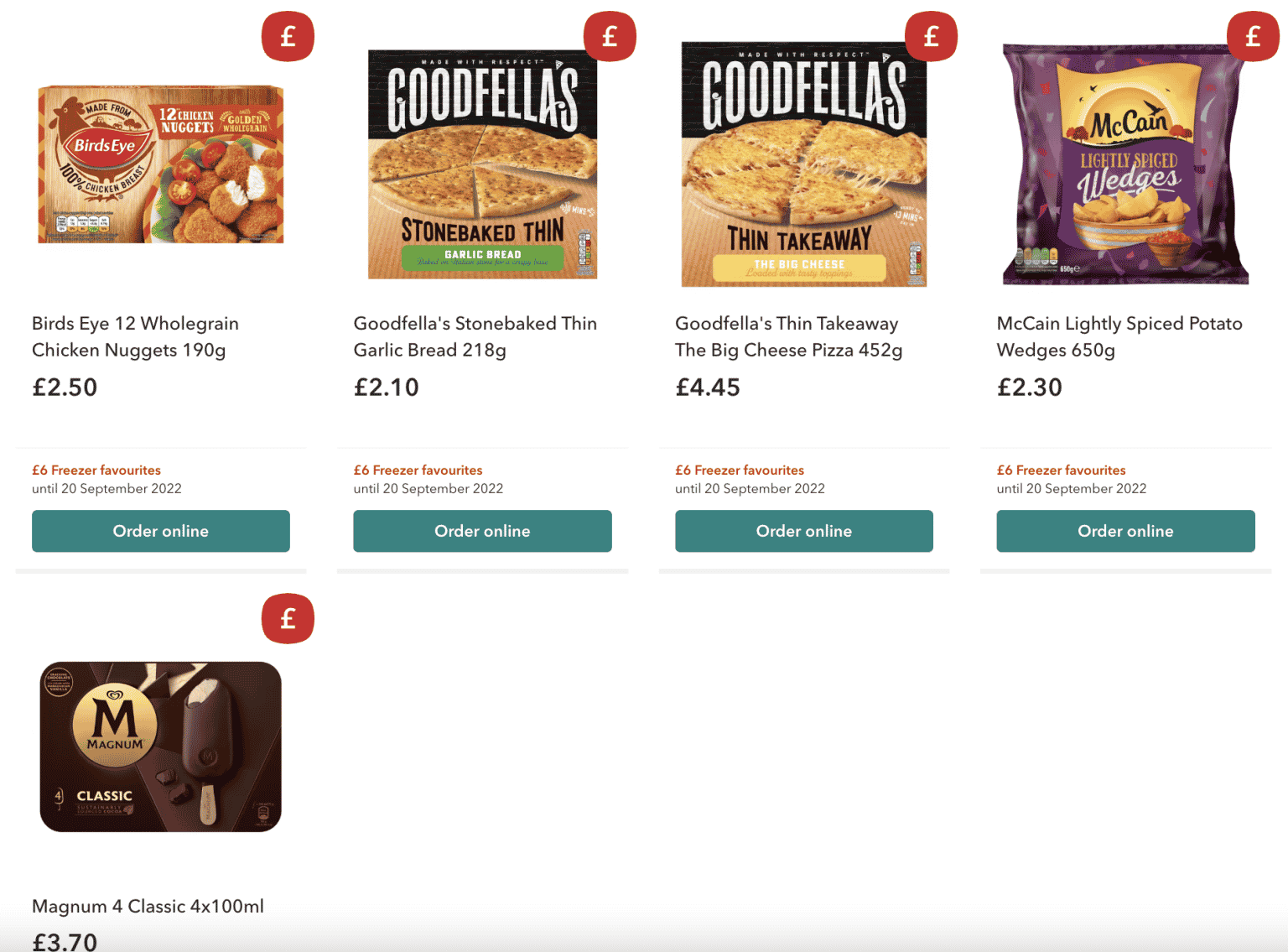**Image Caption of a Food Ordering Website:**

The screen grab showcases a food ordering website with various frozen food items displayed for sale. 

1. The first item is a box of **Birdseye 12 Whole Grain Chicken Nuggets** weighing 190 grams. The nuggets are pictured on a plate, featuring a brown coating, accompanied by slices of red tomatoes and green lettuce. The packaging has a chicken logo and the name "Birdseye" in black font. The price is £2.50. Additionally, there is an orange label stating "Six Pound Freezer Favorites until 20th of September 2022" alongside a teal box with white font indicating the option to order online.

2. The second item is a **Goodfellas Stone Baked Thin Garlic Bread**, weighing 218 grams. The packaging displays the name "Goodfellas" in white on a black background, with the garlic bread resting on a tan surface. This item is priced at £2.10. An identical promotional label to the first item indicates the freezer favorites offer is still valid until September 20, 2022.

3. The third item is a **Goodfellas Thin Takeaway Big Cheese Pizza** weighing 452 grams. The packaging features the "Goodfellas" logo in white, with an image of a cheesy pizza with melted orange cheese. It has a black thin takeaway label beneath the pizza image and a gold box with white font. The price of this pizza is £4.45.

4. The fourth item is a bag of **McCain Lightly Spiced Potato Wedges**, weighing 650 grams. The bag is primarily purple with the "McCain" logo in gold. It depicts an image of potato wedges in a blue and orange bowl, with some illustrations of orange trees and black birds flying in the background. The price for the wedges is £2.30. Similar promotional and ordering details are presented as in the previous listings.

5. The last item is a pack of **Magnum Four Classic Ice Cream Bars**, each 100ml. The packaging has a chocolate brown background with a gold "M" logo. It features an image of the chocolate-covered ice cream bars on sticks. The pack is priced at £3.70.

All items prominently feature the same "Six Pound Freezer Favorites until 20th of September 2022" promotion and have teal order online labels for ease of purchase.